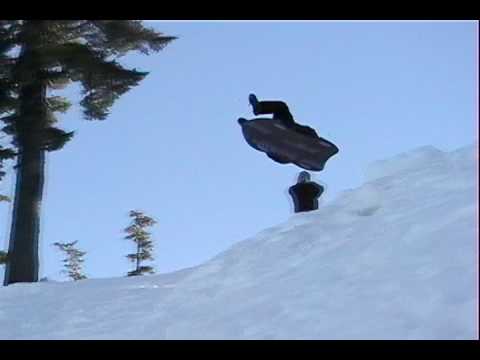The photograph captures an exhilarating action shot of a person on a black sled, mid-air as they soar over a snow-covered hill. The image is taken from a low angle, looking up, emphasizing the height and dynamism of the jump. The sledder, dressed in black, appears to have launched themselves off the snowy hill with their legs outstretched to the side of the sled. Accompanying them is another individual, also dressed in black, positioned to the right and seemingly filming or photographing the airborne sledder. Dominating the left side of the image is a tall brown tree with green leaves. The background features additional trees, adding to the wintry landscape. The overall scene is set during the daytime, providing clear visibility and contributing to the vibrant, energetic atmosphere of the photograph.